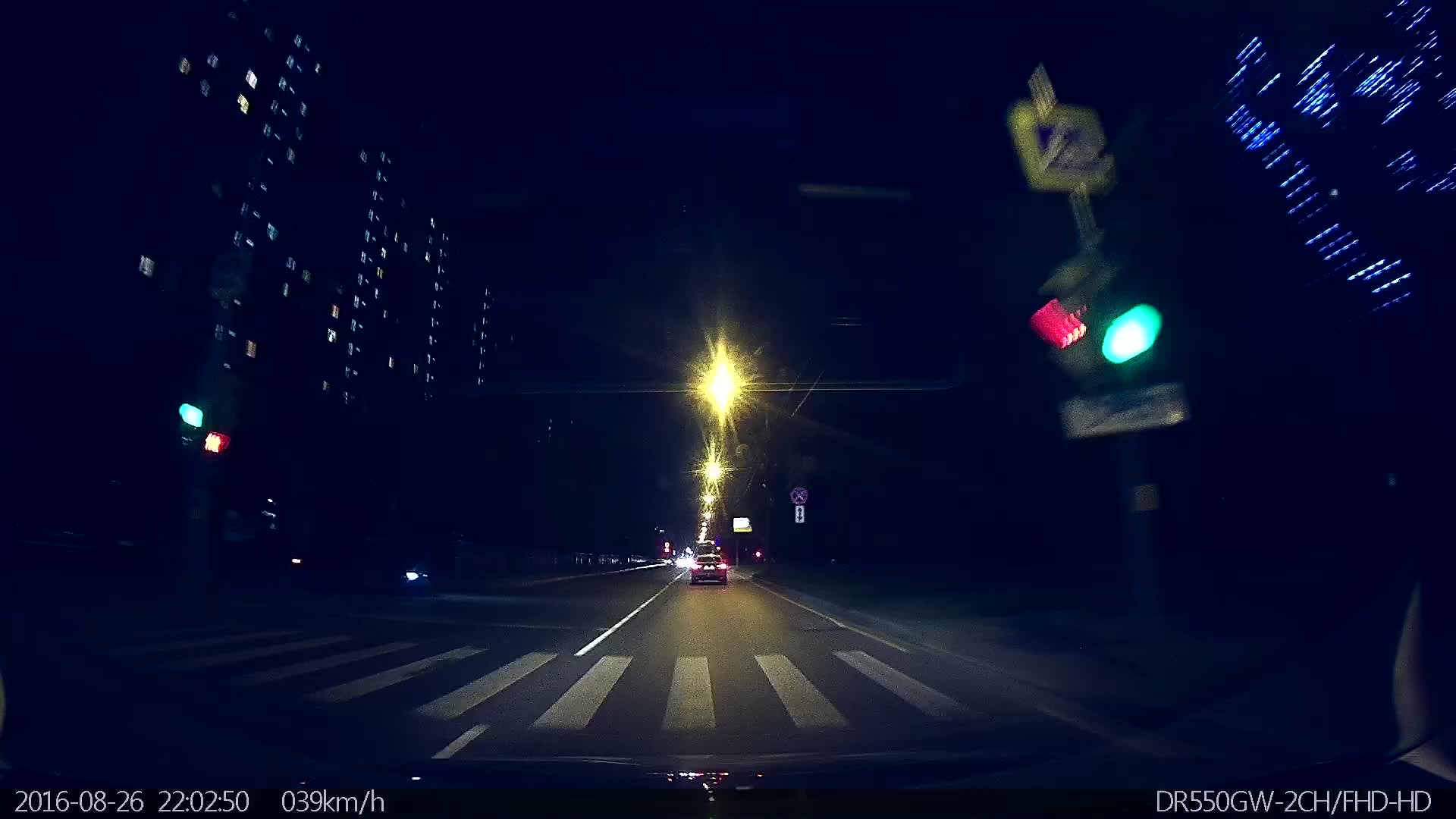This photograph captures a nighttime city scene with a car driving towards the camera, its headlights piercing through the darkness. The image has a slow exposure effect, which creates a striking visual where the streetlights overhead resemble yellow flashes of stars in the sky. The bottom left corner of the photo displays a timestamp that reads "2016-08-26 22:02:50" along with the car's speed, "039 KM/H." The approaching vehicle is nearing a crosswalk, flanked by tall buildings on either side. The buildings, though largely featureless, are dotted with small, scattered lights emanating from their windows, adding to the ambiance of an urban night.